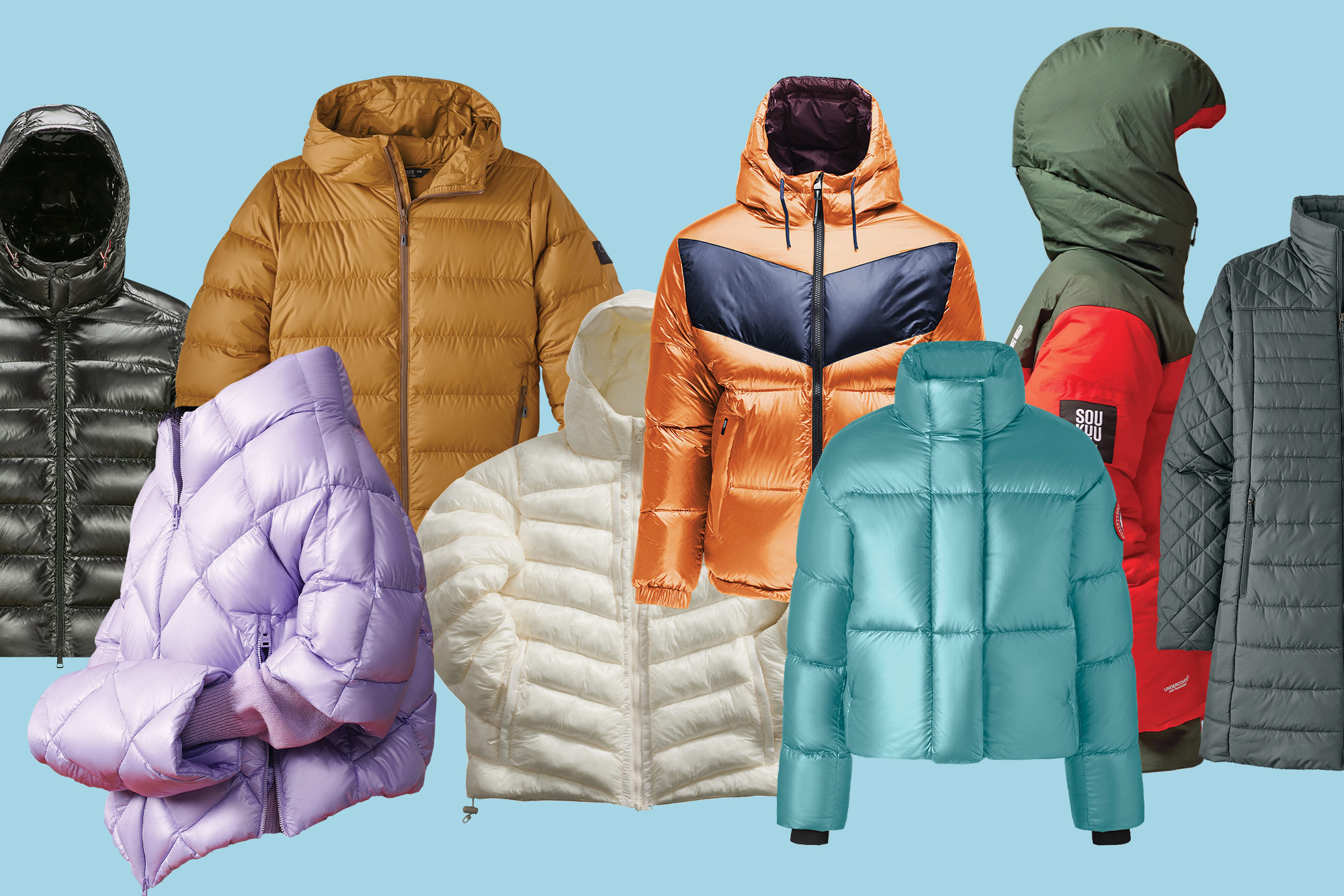This image is an advertisement showcasing a collection of eight different winter coats, all displayed against a sky-blue backdrop. From left to right, the array of puffer jackets includes: a black puffer jacket; an angled purple puffer jacket with hand mitts; behind it, a tan puffer jacket; an off-white hooded puffer jacket; an orange puffer jacket with a hood featuring a broad black stripe across the chest; a teal puffer jacket with no hood; an orange jacket viewed from the side, with a green hood; and partially visible on the far right, a three-quarter length gray puffer jacket. The image features no people or body parts, allowing the focus to remain entirely on the variety of winter coats.